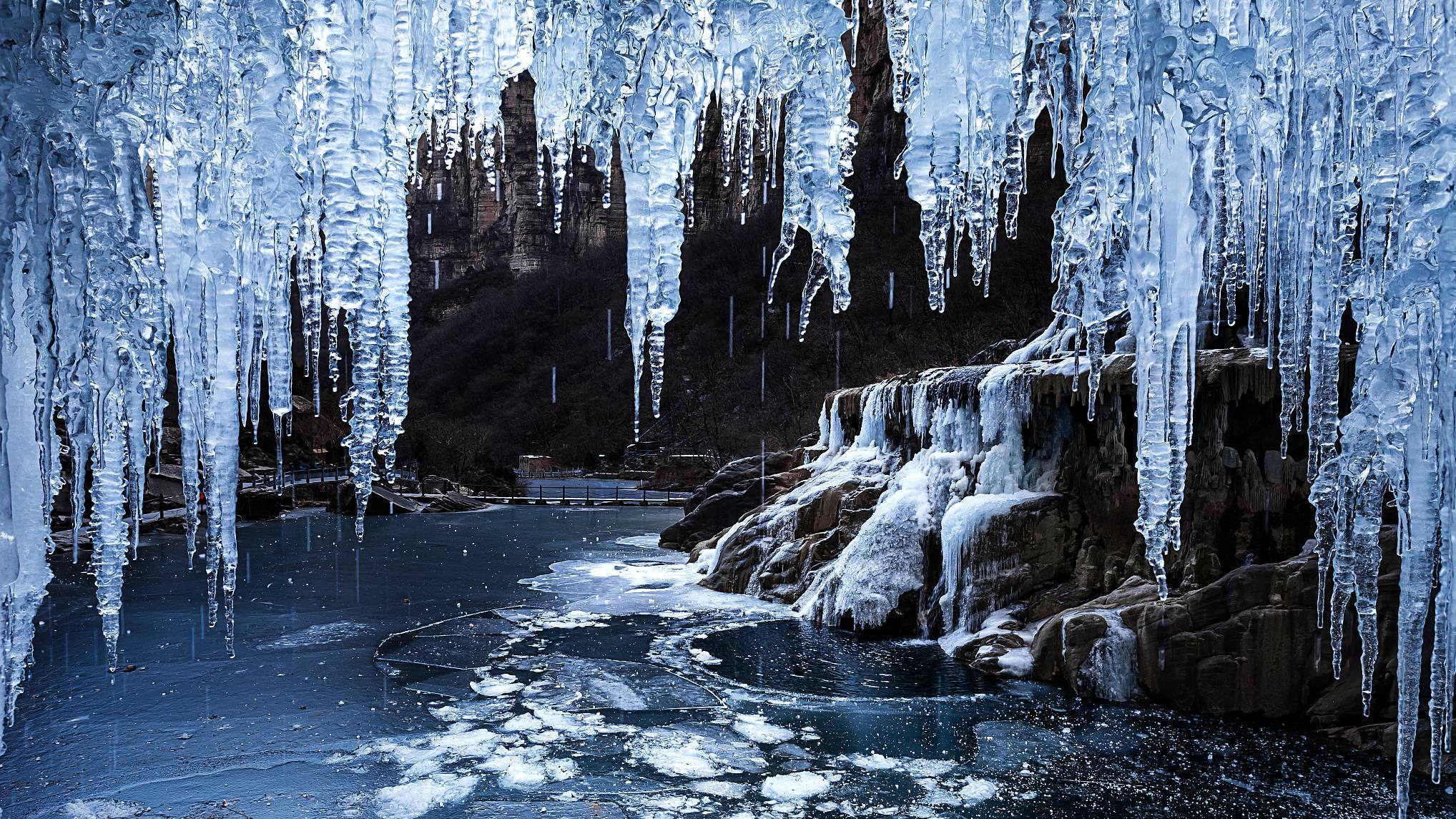This landscape photograph captures a breathtakingly serene and cold scene dominated by enormous, bright blue, dark blue, and pristine white icicles hanging from the top of the image all the way down to a frozen lake below. The background is a deep, almost black expanse that magnifies the striking icicles, which appear to be melting slightly, dripping into the icy, dark blue water. The water, visible more towards the left and right lower corners, interacts with brown rocks and adds a raw, natural element to the otherwise icy tableau. A small bridge and tiny buildings are faintly visible in the distance amidst a leafy, tree-covered mountain, adding depth to the scene. Snow cascades over the rocks on the right, further enhancing the frozen, jagged beauty of the park-like setting. The overall atmosphere is one of serene stillness, slightly warmed by the subtle melt of the icicles.